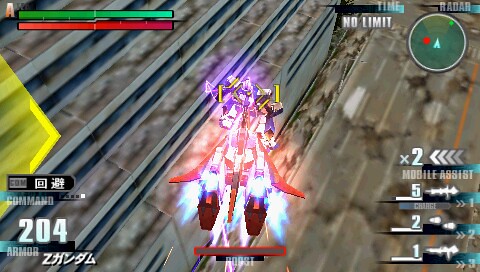This screenshot is taken from an immersive video game. Dominating the center of the frame is the player's spaceship, which features a striking design characterized by a vivid red front, a sleek black rear, and vibrant blue flames trailing from its thrusters. The spaceship's angular, pointed structure exudes a sense of speed and agility. The vessel’s yellow crosshairs are locked onto a target on the ground, a stationary machine or robot colored in white and purple, creating a stark contrast against the terrain. 

The heads-up display (HUD) frames the action, providing crucial information to the player. The top left corner displays two fully filled bars, one green and one red, likely indicating health and shields. Opposite, in the top right, "No Limit" is prominently displayed above a circular radar or map, which positions the player as a central triangle surrounded by small dots representing enemies. Additional HUD elements populate the bottom corners, showcasing numerical data and various indicators labeled with terms such as "Command Armor" and "Mobile Assist," which further enrich the gameplay experience.